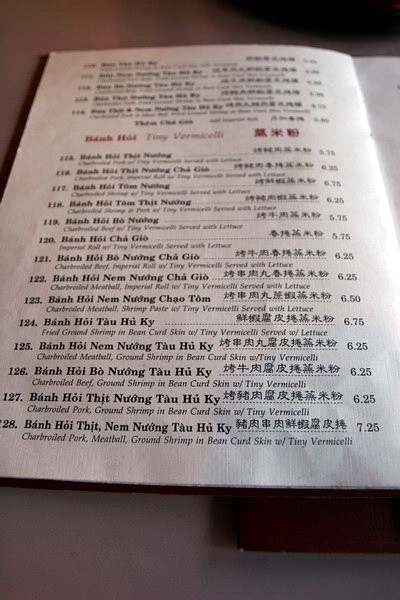The image features a background that transitions from a grayish surface at the bottom to a reddish-brown hue at the top, with darker black accents concentrated in the top right corner. At the center of the photo is an open menu, though only the left-hand page is fully visible. The menu content appears to be written in Vietnamese, accompanied by Chinese characters and an English translation of each dish's ingredients. While the top portion of the menu is blurry and indistinct, the numbers 119 to 128 are clearly visible. The corresponding Vietnamese dish names are followed by their descriptions in English. Prices for the items range from $5.75 to $7.25, although these too become increasingly hard to read towards the top.